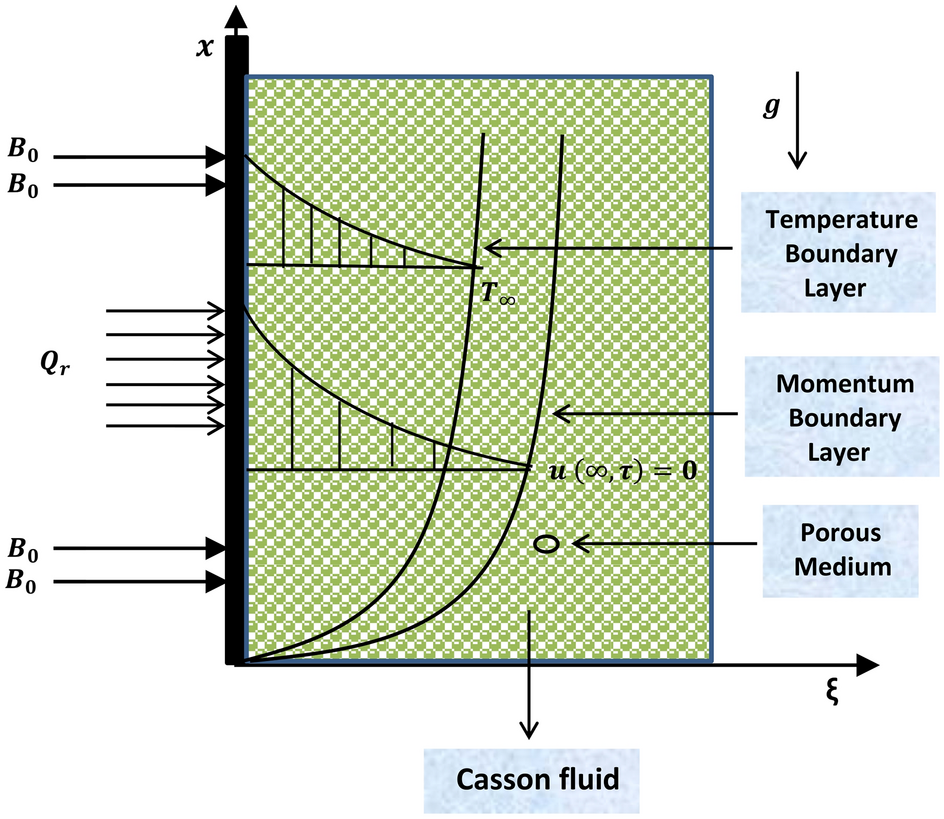The image depicts a detailed scientific diagram with a Cartesian coordinate system, featuring x-axis and eta-axis. The diagram is dominated by a large, rectangular shape intersected with a variety of arrows and lines. The x-axis shows multiple arrows, comprising about four large ones and five smaller ones. To the left, there are labels that read B0, B0, QR, B0, and B0, while the right side features labels such as G (with a downward arrow), temperature boundary layer, momentum boundary layer, and porous medium—all written in black text against light blue backgrounds.

In the center of the diagram is a graph that portrays two distinct curves: a parabolic curve and a downward-sloping curve. The background of the image is white, accented by green bead-like structures, associated with the label "caisson fluid," which is presented in a blue text box at the bottom center of the diagram. Near the middle, an equation is displayed, stating "μ (∞ to τ) = 0." The entire setting is styled comprehensively to represent a scientific diagram, although elements like arrows, triangles, and green structures might make it visually complex.